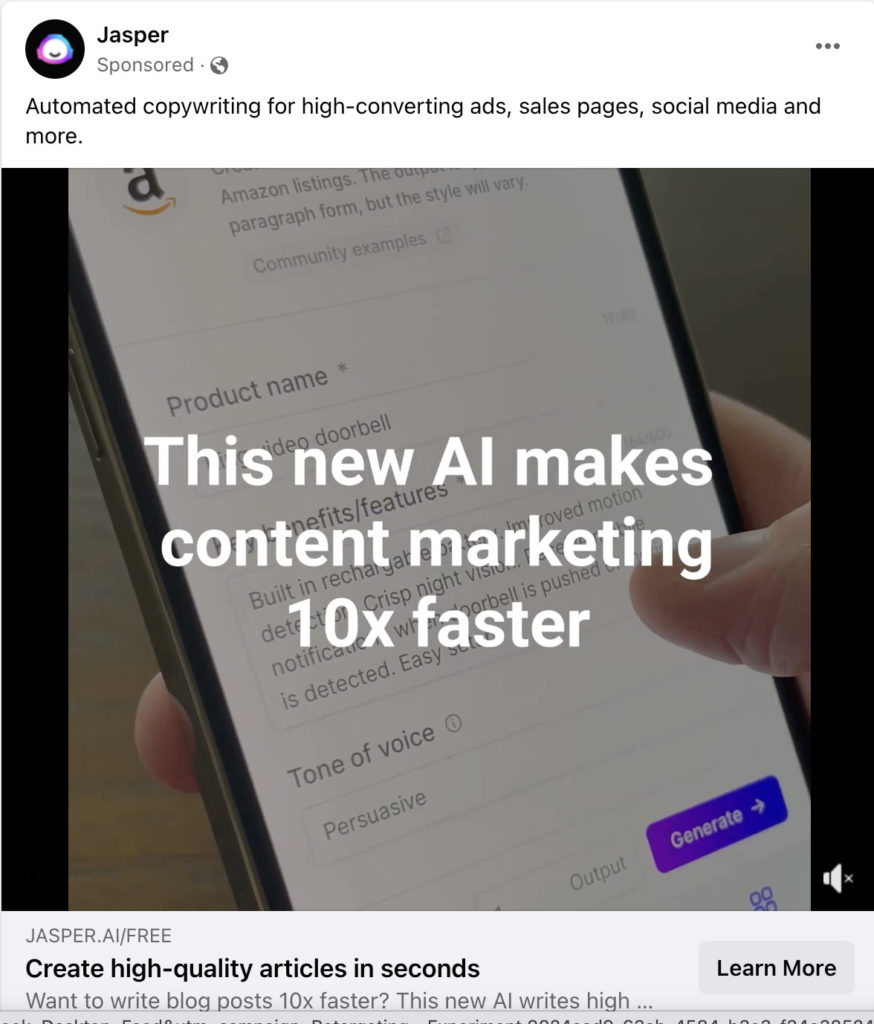Here's a detailed and cleaned-up descriptive caption for the image:

The image features a design predominantly in white, black, purple, pink, and light blue colors. At the top of the image, there is a large white space with a central black circle. Surrounding this black circle, there are concentric circles in shades of purple, pink, and light blue. A curved black line resembling a smile (but not a full smiley face) is superimposed on the larger white area.

Next to this graphic, the word "JASPER" is prominently displayed in black text. Below "JASPER," the word "SPONSOR" is written in gray. Further down, the text "AUTOMATED" appears in capital black letters, followed by a copyright symbol. This is immediately succeeded by the phrase "FORHIDE-CONVERTING-ADS-SALES-PAGES-SOCIAL-MEDIA-AND-MORE."

In the upper right-hand corner of the image, three small gray dots are visible, suggesting a menu or options indicator. The background scene looks like a zoomed-in image of a mobile phone screen, with the screen displaying the text:
- "PRODUCT NAME"
- "BENEFITS-FEATURES-TONE-OF-VOICE-PERSUASIVE."

Above this text, in white capital letters, it says "THIS NEWED AI MAKES CONTENT MARKETING TEN TIMES FASTER."

The bottom section of the image has a gray background where "JASPER.AI-FREE" is written. Below that, "CREATE HIGH-QUALITY ARTICLES IN SECONDS" is displayed in black, capital letters.

There is also a gray box with the text "LEARN MORE" in black inside it. Beneath this box, another gray text says "WANT TO WRITE BLOG POSTS TEN TIMES FASTER? This new AI writes HIGH..." trailing off with an ellipsis because the remainder of the text is obscured in black.

Unfortunately, the bottom part continues in gray, but is partially cut off and not fully visible.